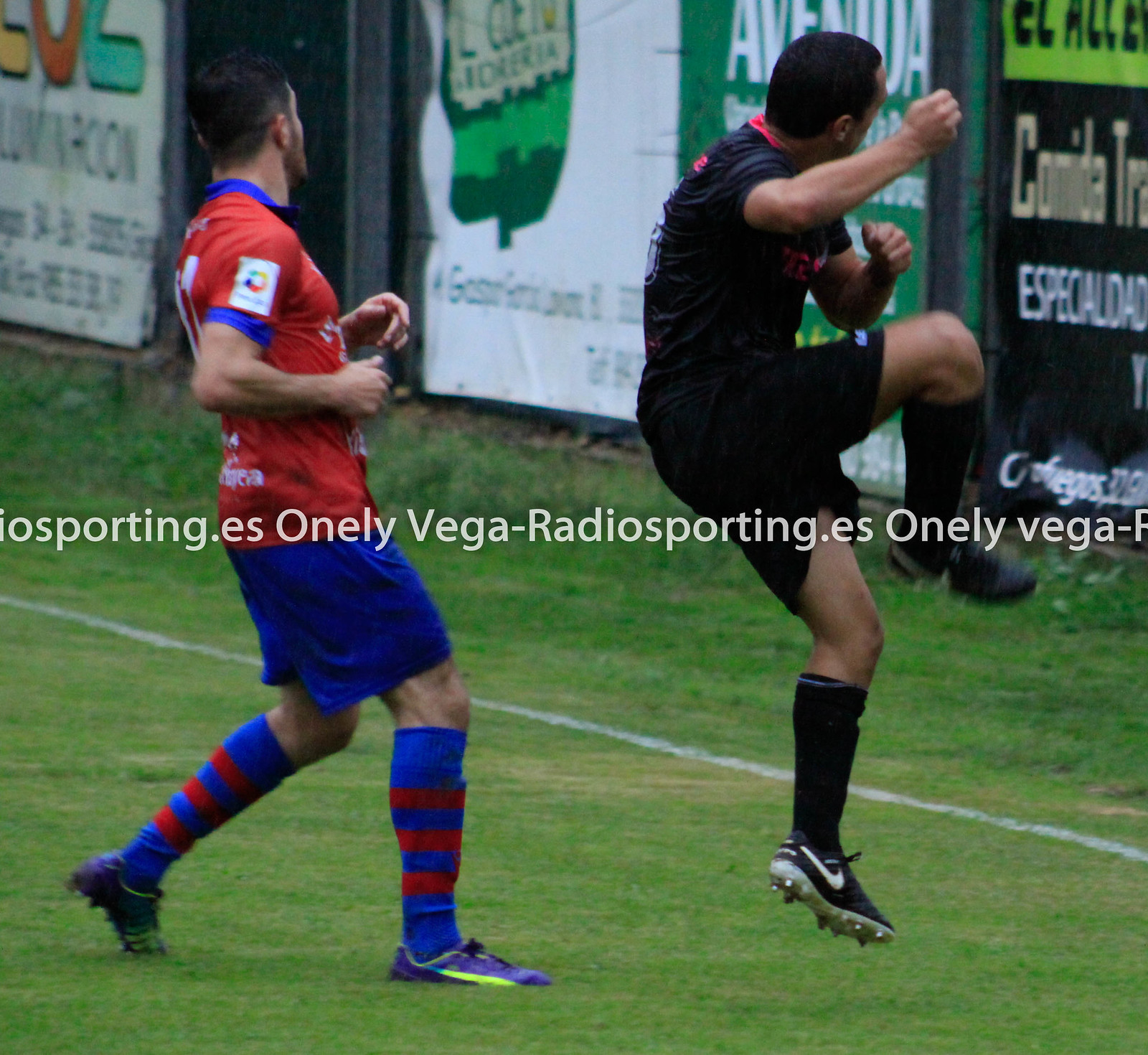The photograph captures a dynamic moment in a soccer match, featuring two players intensely engaged on a vibrant green, grassy pitch, demarcated by a clear white sideline. Both athletes have their backs turned to the camera. The player on the left is clad in an eye-catching red uniform with dark blue shorts, complemented by blue and red striped socks and purple sneakers with yellow stripes. In contrast, the player in black, airborne in the shot, is dressed in a sleek black outfit from head to toe—black shirt outlined with a pink border around the collar, black shorts, socks, and shoes with pink lettering on his back. The backdrop shows a large, blurred wall adorned with four different advertisement banners, partially legible but noticeably containing repeated text that reads "iosporting.es, onlyvega-radiosporting.es, onlyvega." This scene clearly portrays the dynamic and competitive energy of the ongoing soccer match under daylight.